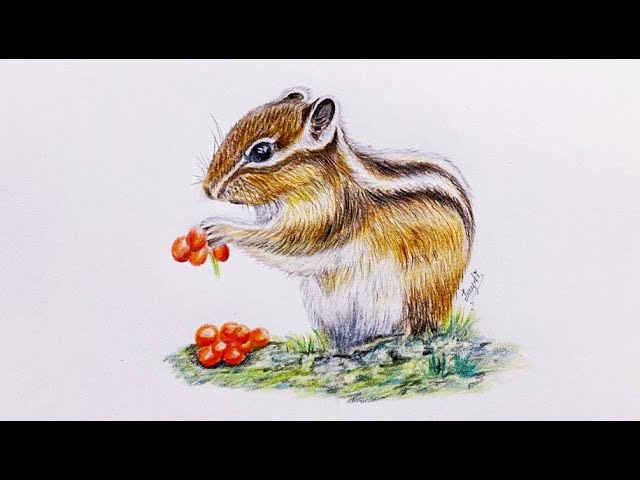The image is a detailed colored pencil drawing of a chipmunk, standing upright on its hind legs and facing left. The chipmunk is holding a cluster of red berries, with more of the same berries scattered in a pile beneath it. The illustration is set against a plain white background and framed by a simple black border at the top and bottom. The chipmunk's fur is intricately textured and artistically rendered with various shades of brown, black, and white, with notable black and white stripes along its back and face. The chipmunk, depicted in profile, showcases its white underbelly and a prominent white stripe running down its back. It has short, perky ears, a stout snout, and realistic whiskers. The ground beneath the chipmunk is a small patch of multicolored, green grass. Despite the precise detailing, the artist's signature is present but too small to read. The overall appearance of the chipmunk is highly realistic and anatomically accurate, capturing the essence of the creature with lifelike detail.